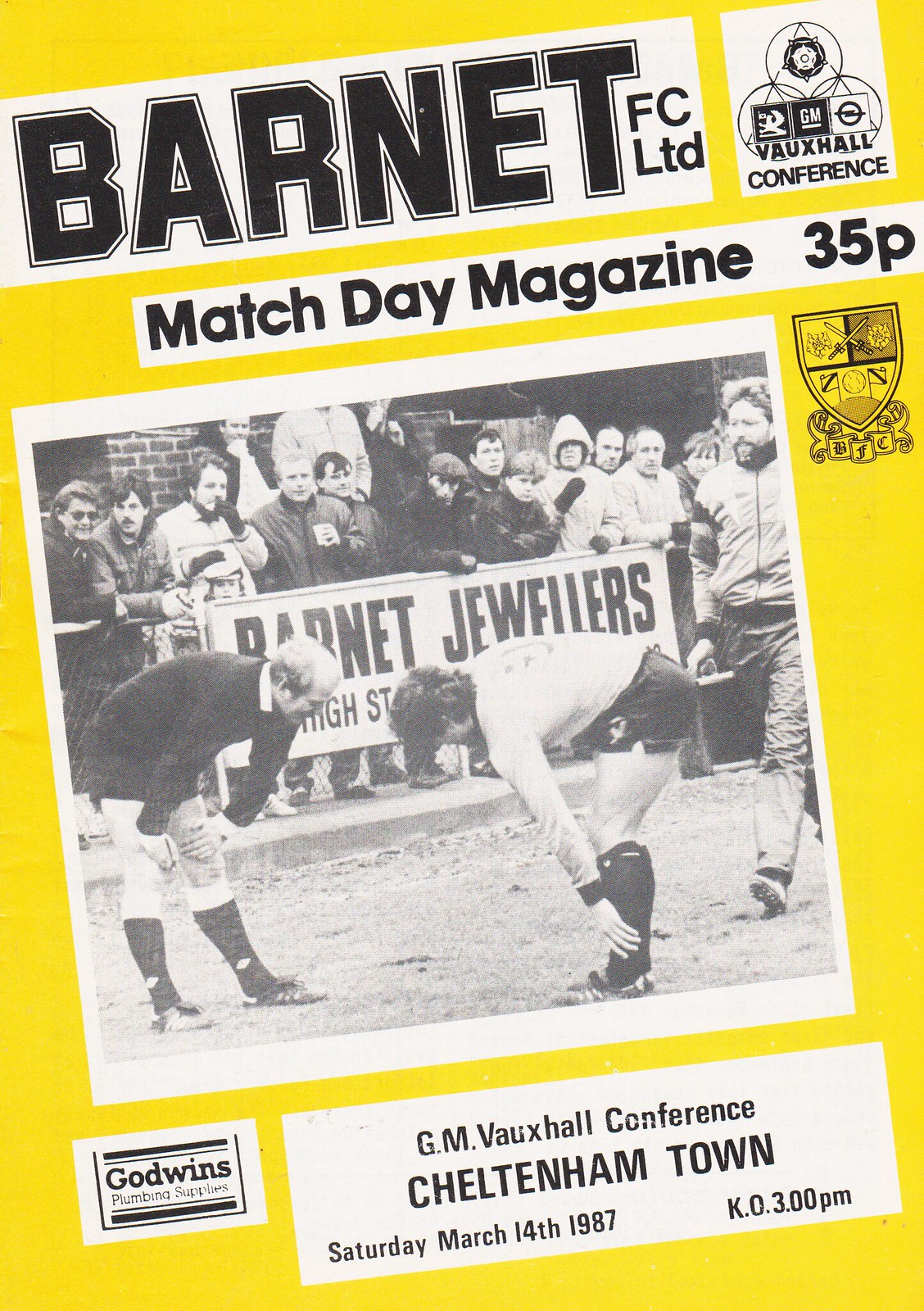The cover of this magazine, boasting a yellow base color, is a striking black-and-white photograph. Titled "Barnet FC Ltd," the magazine is a 35p Match Day publication for a game between Barnet FC and Cheltenham Town, scheduled for Saturday, March 14, 1987, with a kickoff at 3 p.m. The image prominently features two soccer players who are bent over, touching their calves; one player wearing a white top and black shorts, with the other clad all in black, likely the referee. Surrounding the scene are fans in warm coats, indicating chilly weather. These supporters stand behind a prominently displayed sign reading "Barnet Jewelers." In the top right corner of the cover, there's a mention of the GM Voxel Conference. Additionally, on the left side of the cover, there is an advertisement for "Godwins Plumbing Services."